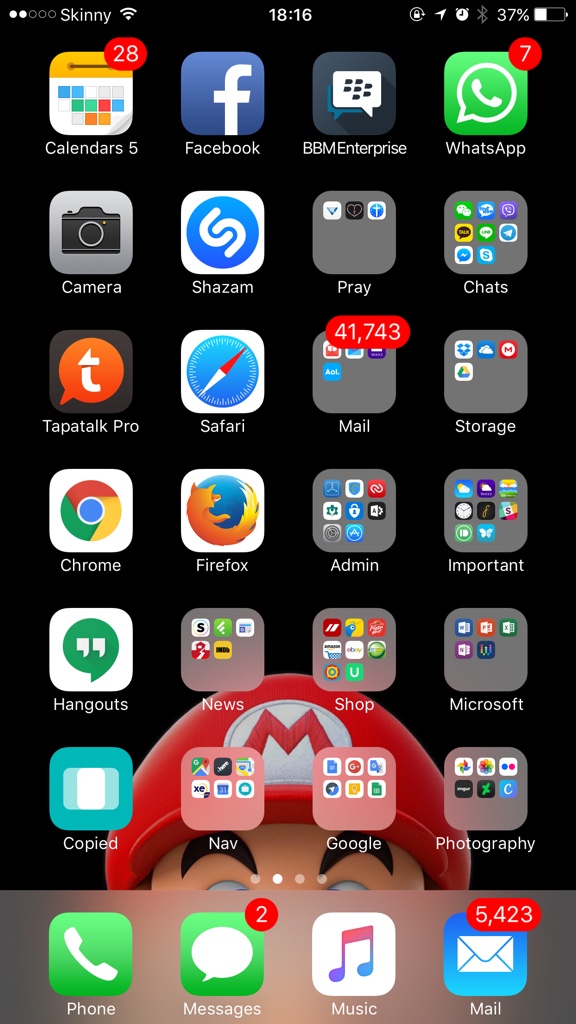In this detailed image of a smartphone screen, various apps and their notifications are displayed clearly. At the top-left corner, the name "Skinny" is visible next to a Wi-Fi signal indicator. Centered at the top, the clock shows the time as 18:16. To the right, icons for Bluetooth, an alarm clock, and a battery indicator showing 37% are displayed.

The main screen beneath this status bar showcases a grid of app icons arranged in a 4 by 7 layout. Starting from the top-left and moving left to right, then downward, the apps are as follows:

- **Calendars 5**: Showing 28 notifications in red.
- **Facebook**
- **BBM Enterprise**
- **WhatsApp**: Indicating 7 notifications with a red circle.

The second row from the top features:
- **Camera**
- **Shazam**
- **Prey**
- **Chats**

In the third row, the apps are:
- **Tap a Talk Pro**
- **Safari**
- **Meal**: Displaying a staggering 41,743 notifications.
- **Storage**

Fourth row:
- **Chrome**
- **Firefox**
- **Admin**
- **Important**

Fifth row:
- **Hangouts**
- **News**
- **Shop**
- **Microsoft**

Sixth row:
- **Copied**
- **Nav**
- **Google**
- **Photography**

In the final row, the apps are:
- **Phone**
- **Messages**: With 2 notifications.
- **Music**
- **Meal**: With another significant number of notifications, totaling 5,423.

This comprehensive layout provides a clear view of the user's most-accessed applications along with their corresponding notifications.